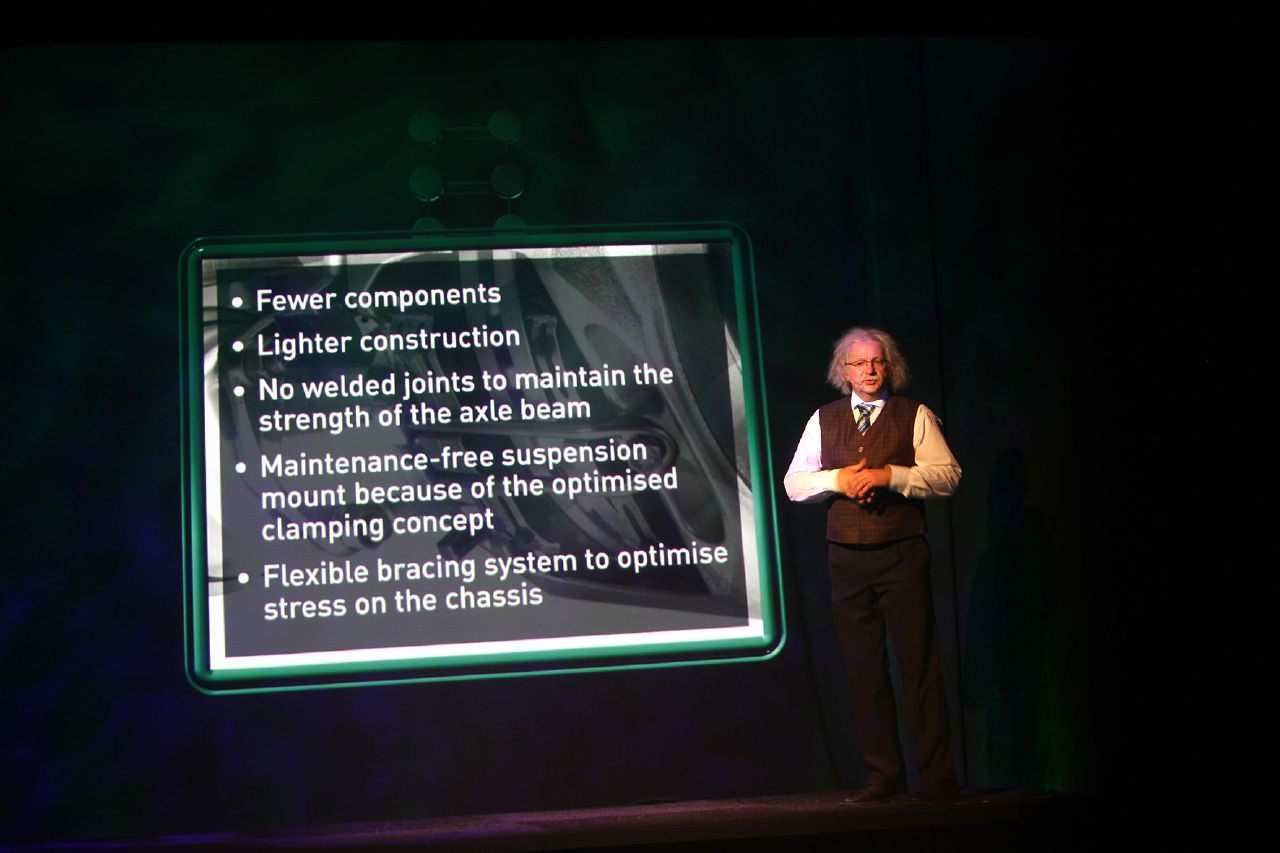In this image, a man resembling Albert Einstein is standing on a stage, presenting next to a projection screen with a green border. He has long, curly gray hair, glasses, and a small goatee. The man is dressed in a brown vest over a white collared shirt, paired with a gray, yellow, and blue tie, black pants, and black shoes. The presentation slide on the screen, which has a green and blue background, features bullet points in white text, highlighting "fewer components," "lighter construction," "no welded joints to maintain the strength of the axle beam," "maintenance-free suspension mount because of the optimized clamping concept," and "flexible bracing system to optimize stress on the chassis." The overall setting is somewhat dark, emphasizing the illuminated screen and the presenter.